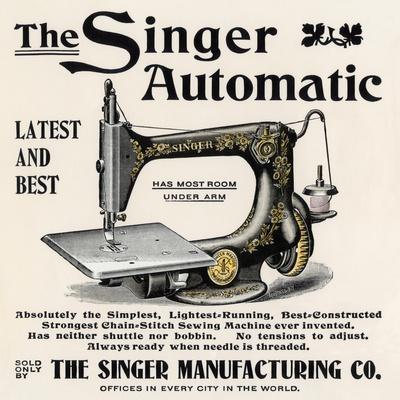The image is a vintage advertisement for the Singer Automatic sewing machine, characterized by a cream-colored background and black lettering. At the top, in elegant fonts with decorative leaf elements, it reads "THE SINGER AUTOMATIC". Below, on the left side, "LATEST AND BEST" is prominently displayed. The bottom section features detailed black text proclaiming the machine as "ABSOLUTELY THE SIMPLEST, LIGHTEST RUNNING, BEST CONSTRUCTED, STRONGEST CHAIN STITCH SEWING MACHINE EVER INVENTED." It highlights key features such as having "NEITHER SHUTTLE NOR BOBBIN" with "NO TENSIONS TO ADJUST", and that it is "ALWAYS READY WHEN NEEDLE IS THREADED."

The ad declares that the machine is sold only at "THE SINGER MANUFACTURING CO. OFFICES IN EVERY CITY IN THE WORLD." Centrally placed is a detailed hand-drawn illustration of the Singer Automatic, featuring a black body with gold patterns and a gold wheel, contrasted by gray-silver metal details. Notably, the machine is threaded with light pink thread and features a spacious area under the arm, emphasized by the text "HAS MOST ROOM UNDER ARM." This advertisement conveys the efficiency and advanced design of what it claims to be the best chain stitch sewing machine of its time.